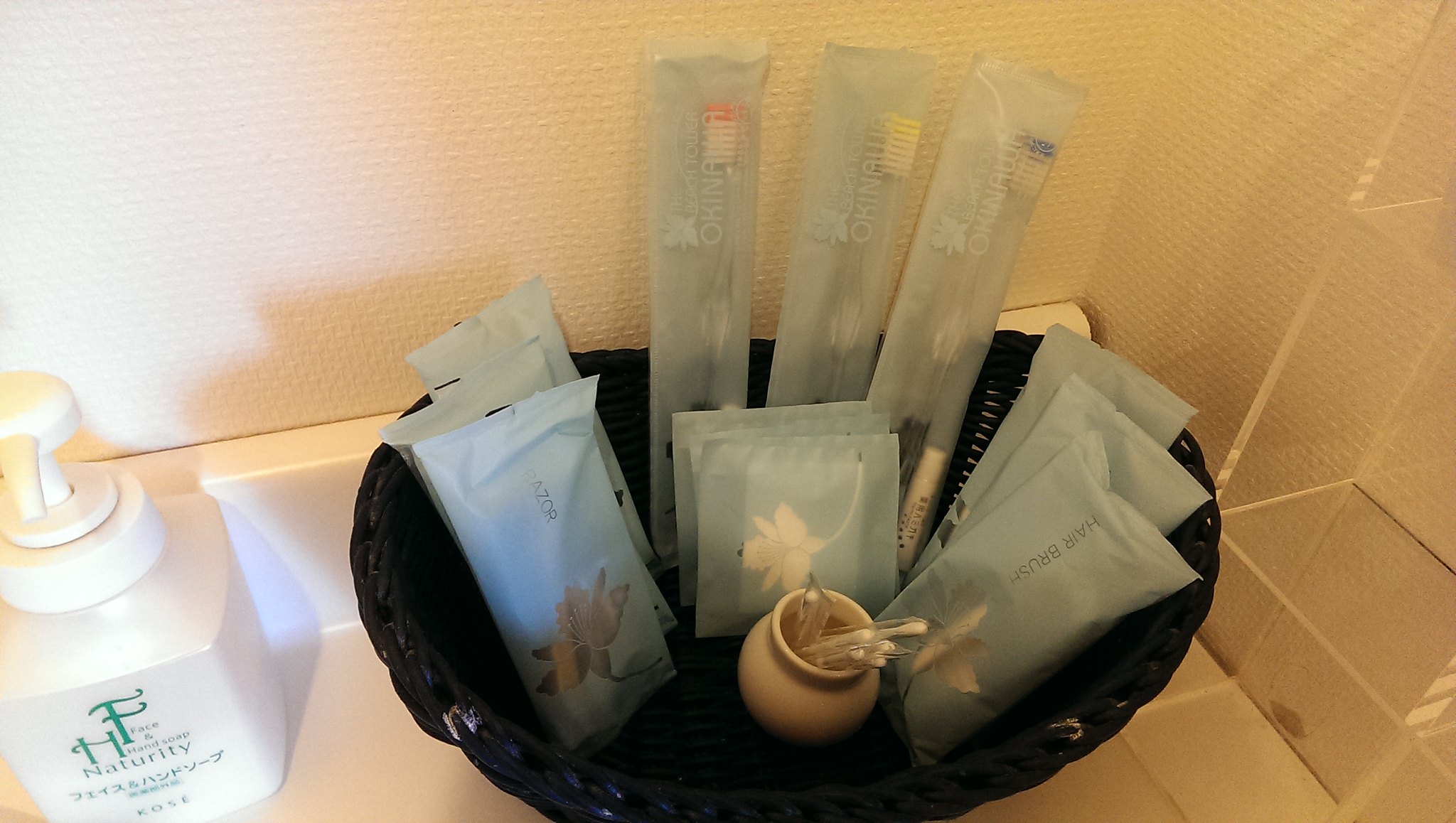The image depicts a bathroom scene, likely within a hotel. Central to the photo is a black, woven basket filled with individually packaged toiletry items. In the basket, we can clearly see at least three toothbrushes—identifiable by their pink, yellow, and blue packaging—alongside razors, tissue packets, and a separate package containing a hairbrush. Additionally, a small pot holds cotton swabs. Positioned to the left of the basket is a white pump bottle of face and hand soap, labeled with the brand "HF NATURITY" and Japanese characters. The soap dispenser features green text on the white bottle. The arrangement sits atop a white countertop, and in the background, a glass partition for a shower stall is partially visible against a white wall.